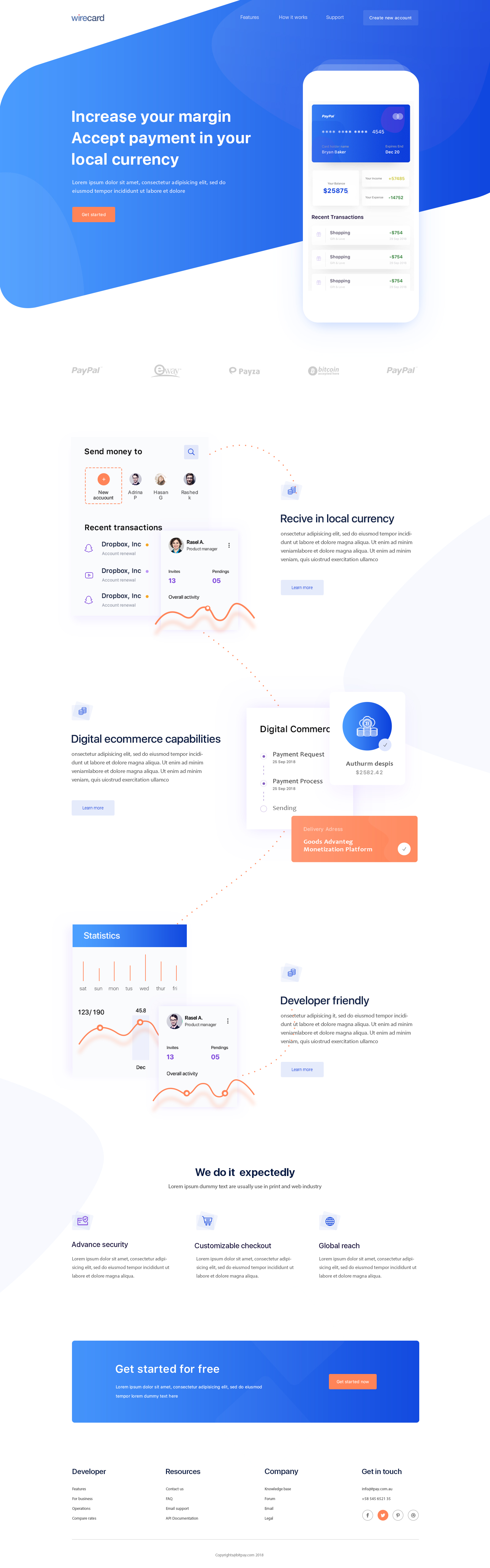The screenshot displays a webpage for Wirecard, which is prominently indicated by the "Wirecard" logo situated in the upper left corner. Directly below the logo is a visually appealing blue banner featuring the text, "Increase your margin, accept payment in your local currency," alongside an inviting orange "Get Started" button.

Within the same blue banner on the right side, there is an embedded screen showcasing a PayPal debit card graphic. This PayPal card is blue with the name "Brian Baker" and an expiration date of "December 2020." The card number begins with "4545," and it indicates a balance of "2,058.75," although the number formatting is somewhat unclear.

Continuing down the webpage, various logos for popular payment platforms such as PayPal, E-Way, PESA, and Bitcoin are displayed, along with another PayPal button. There are also instructions describing the platform's functionality, emphasizing its capability to send money internationally and convert it automatically to local currencies. This section is illustrated with icons representing people and money transactions.

Further down, the page includes numerous promotional sections highlighting the platform's features, such as digital e-commerce capabilities and being developer-friendly. The content emphasizes the website's efficiency and user-friendly nature, making it a robust solution for e-commerce transactions.